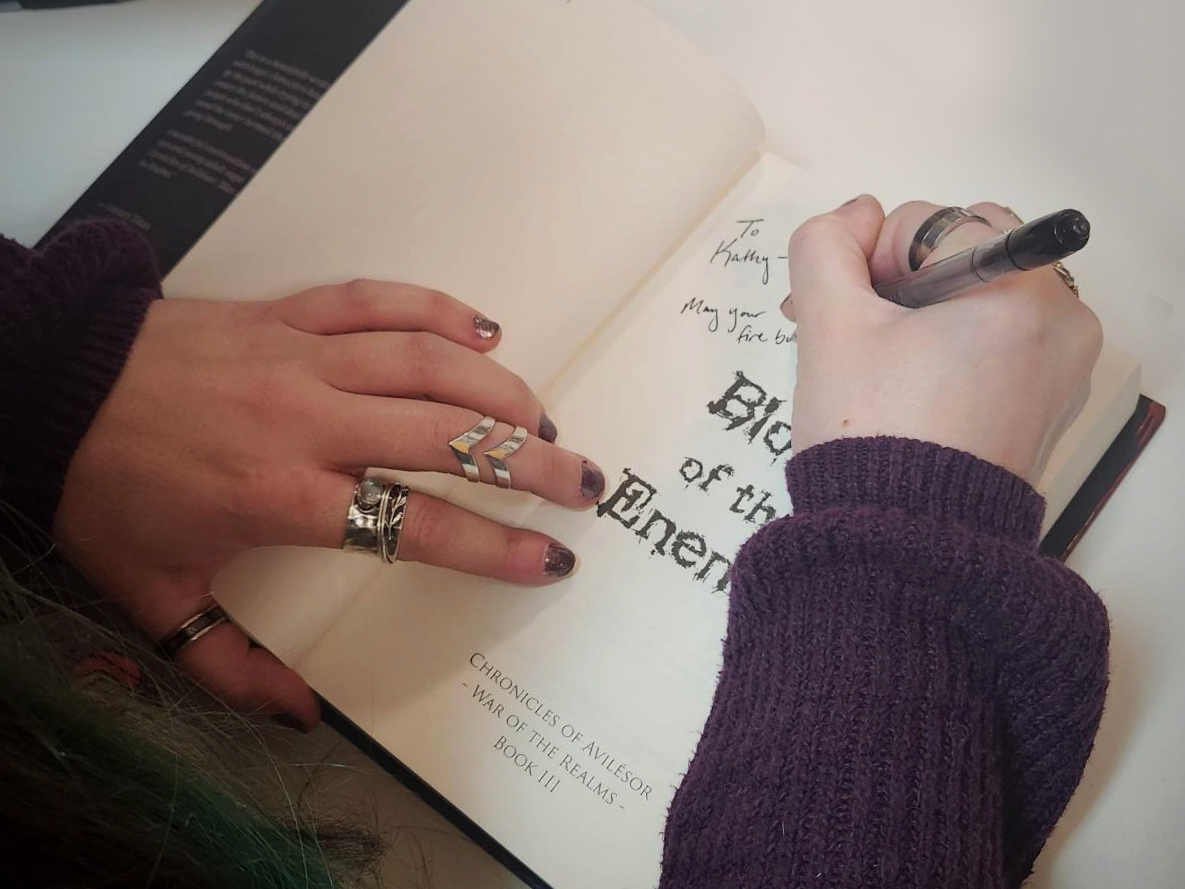The photograph captures a close-up of a woman, presumably the author, signing a copy of "Blood of the Enemy," the third book in the "Chronicles of Avelisir: War of the Realms" series. Only her hands are visible, with numerous silver or platinum rings adorning both her left and right fingers. Some rings include inlaid stones, and she is wearing a metallic, copper-colored nail polish. Her left hand helps keep the hardcover book open, while her right hand, holding a black pen, inscribes a dedication: "To Cathy, may your fire be..." She is clad in a thick purple sweater, and the book rests on a white table, showcasing the title page where the signing takes place.